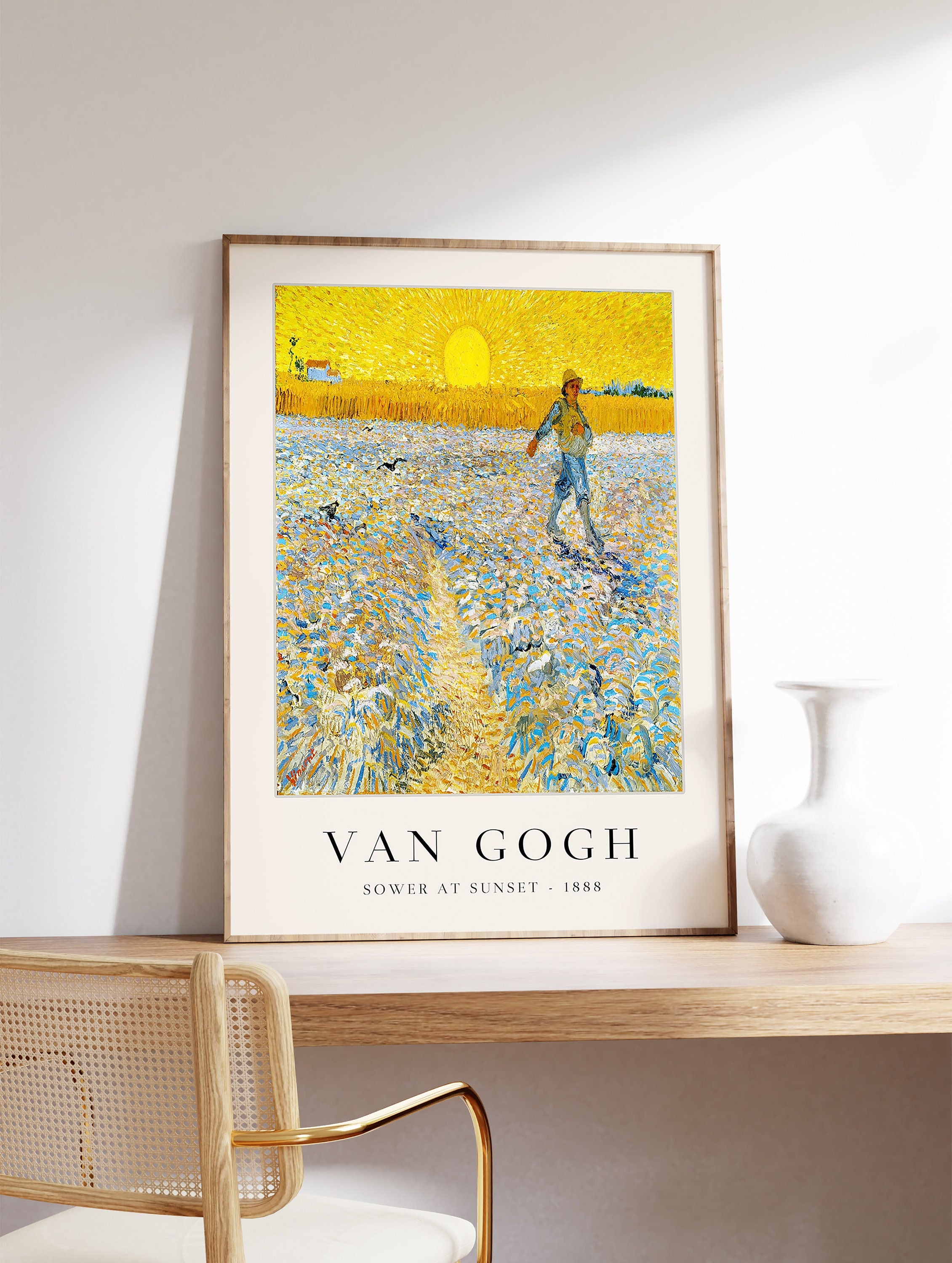The image captures a detailed scene of a 3D color illustration rendered in portrait orientation. At the center of the composition, a framed Van Gogh poster art leans against a white wall on top of a light wood-finished table. The painting itself features a depiction of "Sower at Sunset, 1888," showcasing a figure walking through a field with blue and cream-colored vegetation, birds flying overhead, and a yellow sun setting on the horizon beside a small farmhouse. The poster has the text "Van Gogh" prominently displayed at the top in large black letters, followed by "Sower at Sunset, 1888" in smaller text underneath.

To the right of the painting, a white ceramic vase with a rounded base, tapered neck, and fluted top adds an elegant touch to the scene. The table appears almost to be floating since its legs or supports are not visible, giving it an ethereal feel.

On the bottom left of the table, a wicker chair with a woven cane back and a cushion seat is pulled out slightly. The chair features a cream-colored cane back framed in light wood, with a brass-colored curved arm extending across the right side. Subtle details include small holes in the wicker back. The photo is captured from a slight angle, indicating that the photographer stood off slightly to the left, creating a sense of depth and perspective. The indoor setting of this illustration is apparent, though it remains ambiguous whether the photo was taken during the daytime or nighttime.